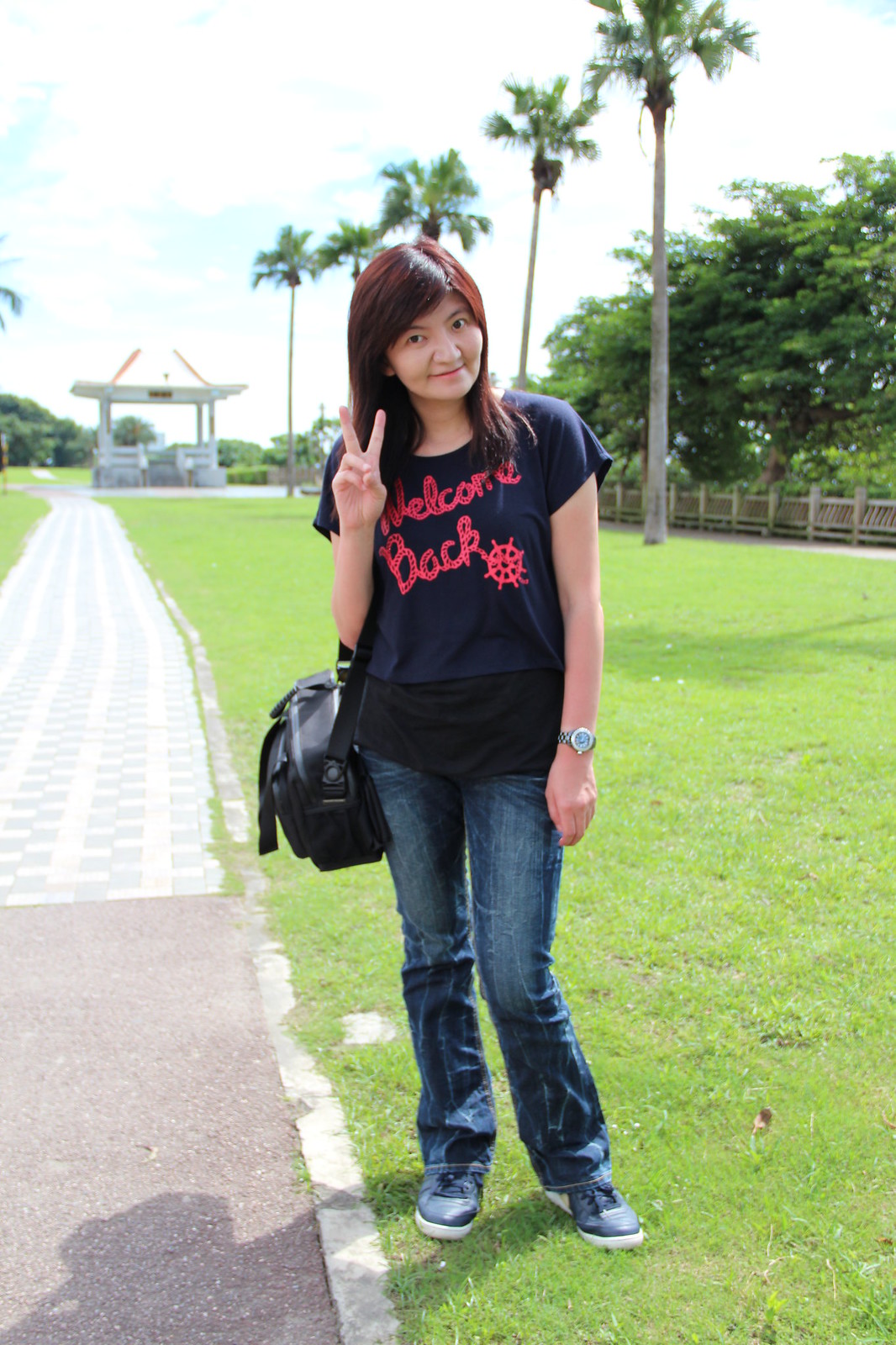In the portrait-oriented color photograph, a young Asian woman, around 25 years old, is standing in the center on a green grassy path with a partially concrete, partially stone pathway beside her. She is smiling and flashing a peace sign with her right hand, which is on the left side of the image. The woman has shoulder-length, dark reddish-brown hair and wears a short-sleeved t-shirt that is black at the top and blue at the bottom, adorned with the words "Welcome Back" in bold pink script along with the symbol of a ship's steering wheel. She accessorizes her outfit with a silver watch on her right wrist, blue jeans, dark blue sneakers with white soles, and a black bag slung over her right shoulder. The background of the image depicts a tropical location with tall coconut palm trees, a wooden fence, and lush greenery. A small concrete structure, such as an arch or overhead canopy, appears along the pathway that leads into the distance. The sky above is bright and slightly cloudy, completing the serene and welcoming scene.